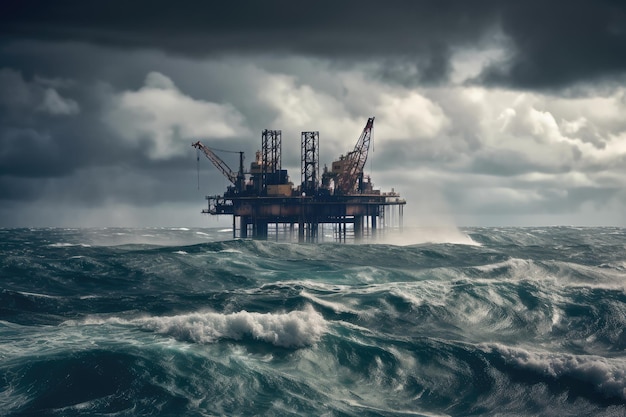This is a striking depiction of an oil drilling rig braving a tumultuous storm in the ocean, possibly the Gulf of Mexico. The ocean is a tumultuous mix of deep blue-gray and greenish-gray waves, capped with foam and mist from their constant churning. The rig stands on numerous tubular pilings, supporting a complex lattice of metalwork, derricks, living quarters, and working areas above the thundering sea. On the left side of the rig, a crane arm extends outward with a wire hanging down, while on the right, another crane faces more towards the back. The sky is dramatic, with a gradient from white clouds near the horizon to ominously dark clouds at the top of the image, contributing to the surreal, almost unreal atmosphere captured in this photograph.